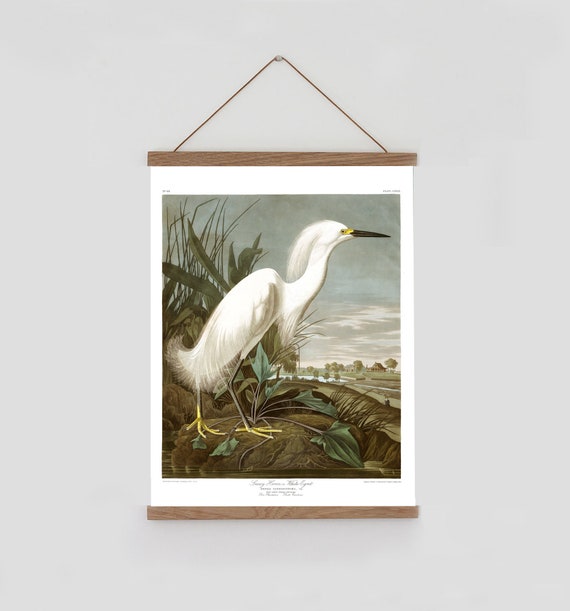This photograph captures a framed illustration hanging elegantly on a light gray wall. The illustration is enclosed in a brown wooden frame, suspended by a brown string that creates a picturesque V-shape at the top, perfectly draped over a central nail. The focus of the illustration is a magnificent snowy heron, depicted with meticulous detail. The heron showcases its striking long, flowing white feathers that cascade like ethereal hair. Its slender, elongated beak is predominantly black with a yellow base seamlessly blending into its face. The bird’s stature is accentuated by its long, black legs and contrasting yellow feet, presenting a poised, graceful stance atop a verdant mound of green grass. The heron is encircled by lush, bright green-leaved plants, with taller, darker green grasses forming the backdrop, creating a serene and naturalistic setting that highlights the bird’s elegance.